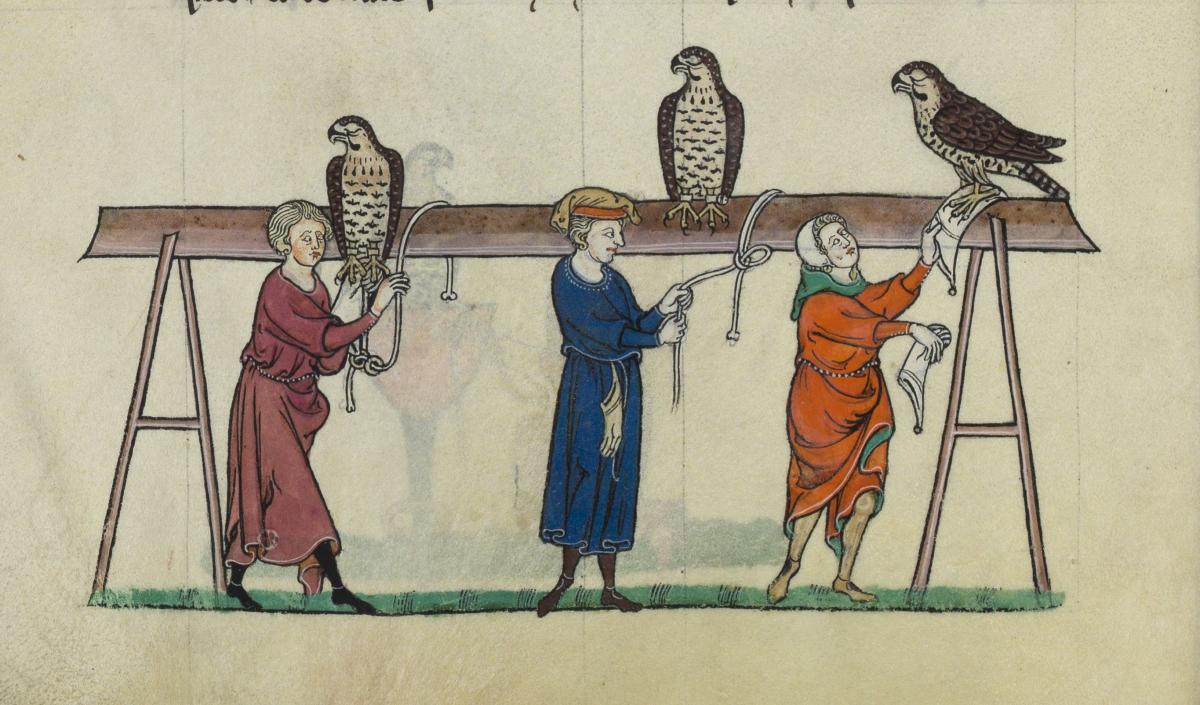This intricate drawing, possibly an old piece of artwork in pencil, colored pencil, or felt pen, features three women tending to birds. The scene is set outdoors, depicted against a slightly dusky white background, hinting at the artwork's age. The women are standing on green grass and are dressed in long, period-specific dresses; their attire includes ropes tied around their waists and bandanas covering their heads.

The central focus is a wooden platform that runs horizontally from the center left to the center right, supported by triangular wooden pegs at each end. Perched on this plank are three large birds, identified as owls in some descriptions and hawks or eagles in others. The birds have tags on their feet, suggesting they are under the care of professional bird handlers. One bird faces forward, another looks to the right, and the bird on the far right is seen in left profile. The women are tying ropes to the platform and attaching something to the birds' talons, perhaps preparing them for flight or securing them in place.

The women’s detailed clothing includes one in a light purple dress with gray hair and black stockings, another in a blue dress with a red or orange bandana over her yellow hair, and the third in an orange dress with a green bandana and barefoot, wearing a little hat. The faded, blurred background elements add to the image's historical ambiance, making it reminiscent of artwork one might find in an old English castle.